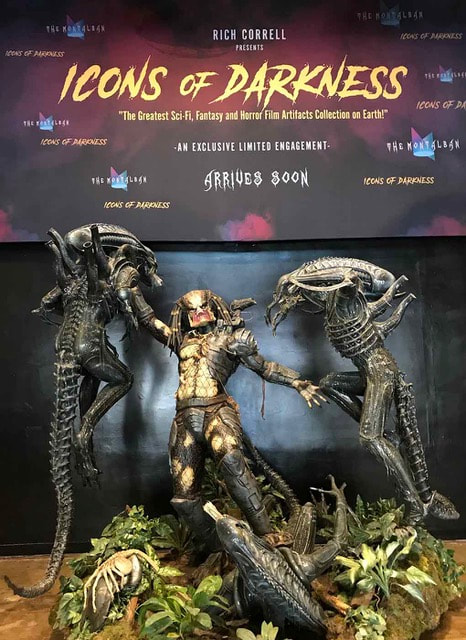This is a detailed poster advertising *Icons of Darkness*, a collection of the greatest sci-fi, fantasy, and horror film artifacts curated by Rich Correll. Dominating the image is a striking scene where a Predator engages in a fierce battle with multiple alien creatures. One alien is pinned under the Predator's foot, while another seems ready to pounce. The aliens, with their long, seahorse-like tails and grotesque features, add a menacing aura to the display. The encounter takes place on a sparsely vegetated plot, with ominous outlines of more creatures emerging in the hazy background. Above the confrontation, the title *Icons of Darkness* is emblazoned in bold yellow, promising an exclusive, limited-engagement exhibition that arrives soon. The vivid imagery of this poster effectively evokes the terror and excitement of these legendary sci-fi and horror icons.